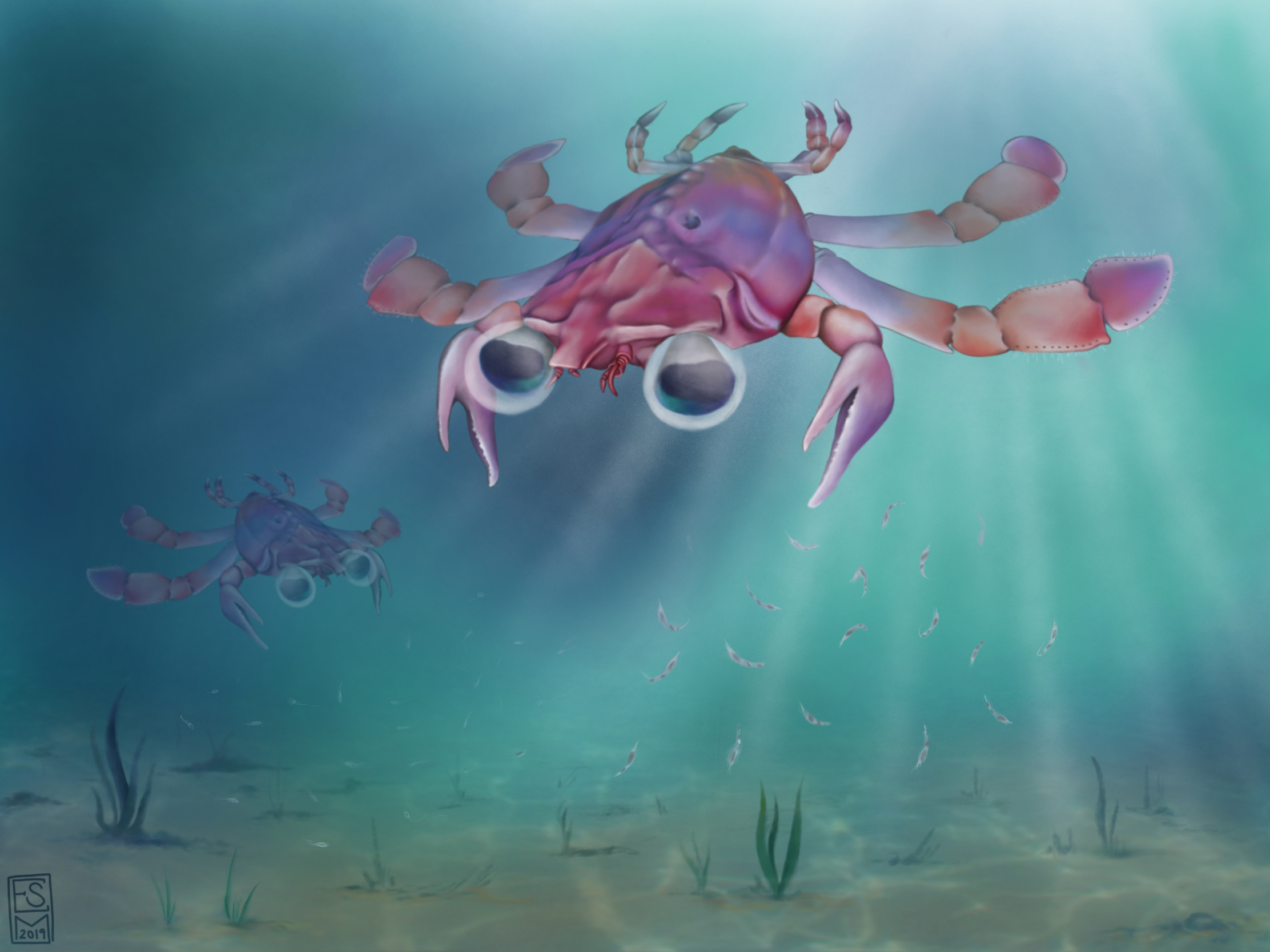The image is a cartoonish, low-detail, 3D depiction of two crabs with exaggerated, bubble-shaped eyes at the bottom of the ocean. It features vibrant colors: the crabs are painted in shades of purple, pink, orange, and lavender. One large crab is prominently displayed in the foreground, showcasing four legs on each side, two large pincers, and strikingly oversized eyes. The second crab, a mirrored version of the first, appears smaller and more blurred in the background. The seabed is flat with sparse, seaweed-like plants scattered around. Sunlight beams filter through the water, creating a contrast between the lighter blue areas where the sun hits and the darker blue shades elsewhere. Tiny shrimps swim around, and a signature reading "S 2019" is inscribed in a vertical rectangle on the lower right side of the image.